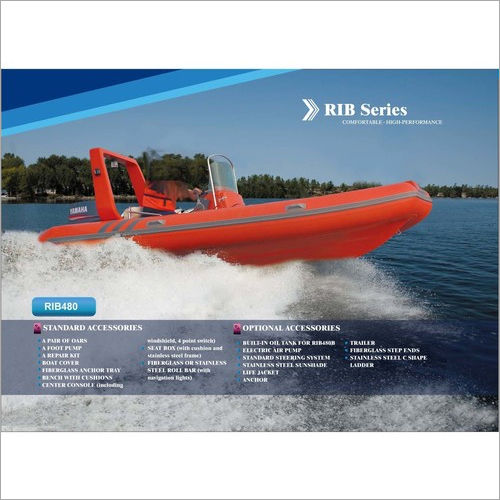This image is an advertisement for a jet boat, prominently featuring an orange speedboat creating waves on a lake. The background showcases a clear blue sky with a line of trees stretching from left to right. In the upper left corner, the advert has three stripes in varying shades of blue: dark blue on the top, medium blue in the middle, and light blue below. The text in the upper right corner reads "RIB Series, Comfortable, High Performance," accompanied by an arrow graphic. Near the center, to the left, there's a blue rectangular box labeled "RIB 480." Below this, a semi-transparent blue box details numerous standard and optional accessories, though some of the text is hard to decipher due to small, white lettering. Featured accessories include a foot pump, repair kit, boat cover, fiberglass anchor tray, bench with cushion, and center console.